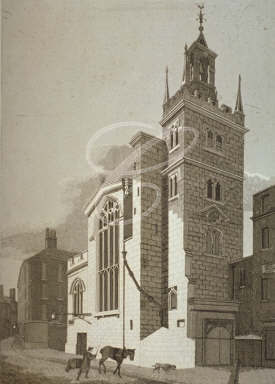The black-and-white illustration depicts a grand, tall brick building reminiscent of a church with a large tower on the right side, crowned with an additional smaller tower that resembles a bell tower, complete with a pointy roof and possibly a weathervane. The building features large, arched cathedral-style windows, along with a set of smaller arched windows on its left side. A road and a sidewalk stretch out in front of the building, with a person leading a horse along the road. Another figure, not entirely identifiable, stands on the sidewalk. In the background, another shorter and darker building with a chimney is partially visible behind the main structure, and to the right of the image. The scene is rendered in shades of gray, giving it a classic, timeless feel. The composition is completed by a cursive "C" superimposed at the top center of the image. Overall, the detailed architecture and elements resemble an old Western town.